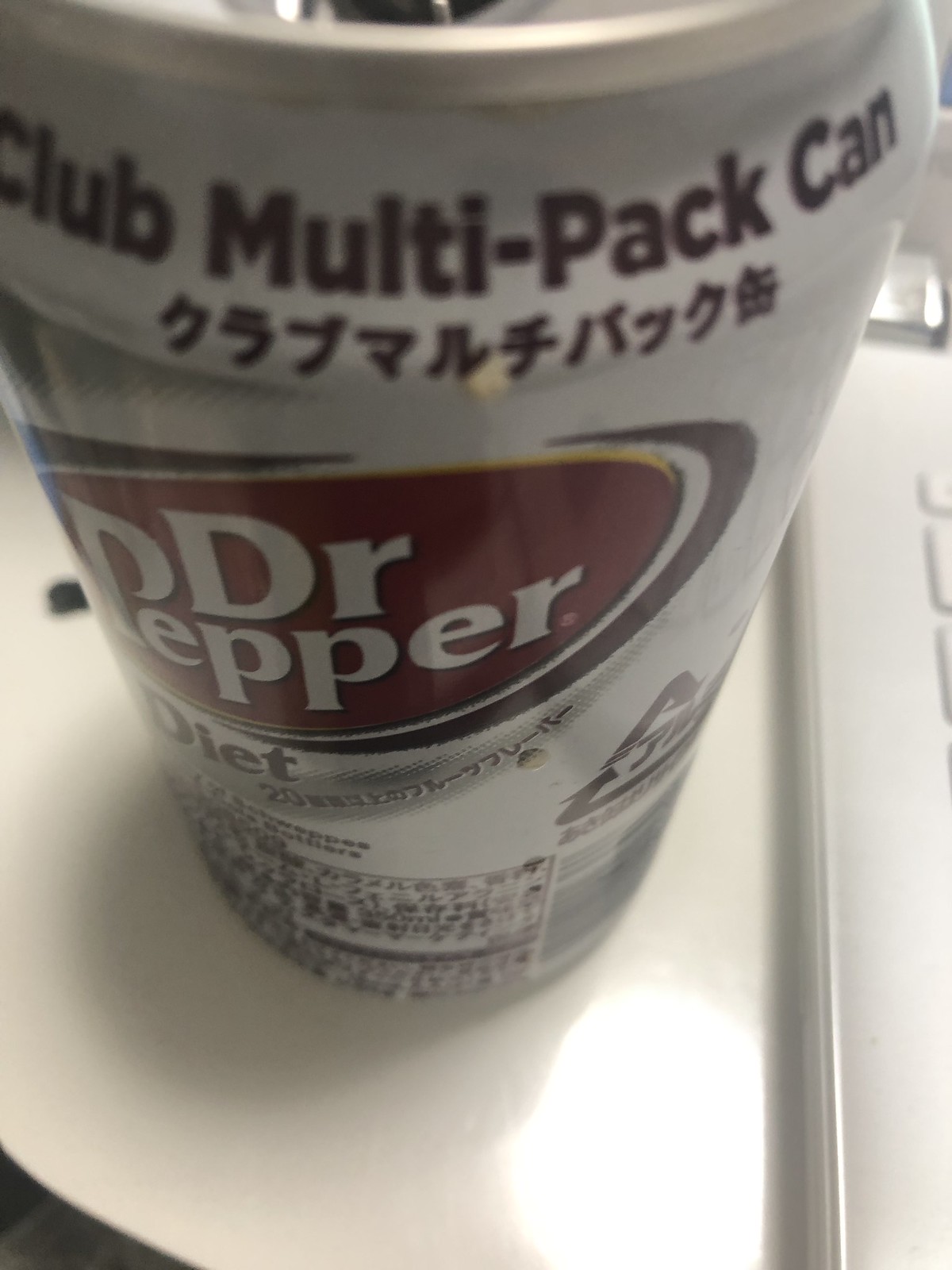A detailed close-up image captures a Dr. Pepper can from a top-to-bottom angle. The primary focus is on the front of the can, which features both English and what appears to be Japanese or Chinese text, suggesting it is an international variant. The can is prominently displayed on a round white table, occupying the majority of the frame. To the right, a portion of a laptop is visible, with some of the keyboard keys and part of the hinge in view, confirming it’s a portable computer. The high level of detail and the objects' arrangement create a cozy, everyday setting.